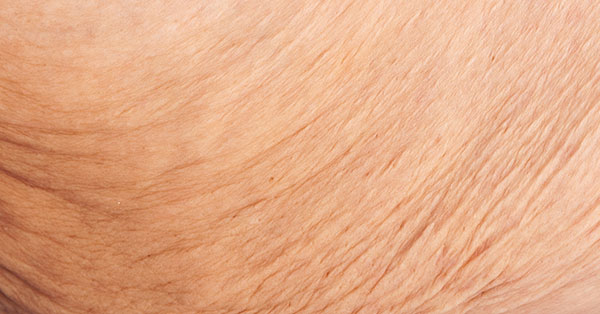This photograph provides a detailed, very close-up view of a patch of heavily wrinkled, light-colored skin, most likely belonging to an elderly, Caucasian individual. The skin is devoid of blemishes, pimples, or visible hair. The texture and heavy wrinkling suggest advanced age, potentially in the 80s or 90s. The image's composition makes it difficult to precisely identify the body part, but the skin's curvature and shadowing hint at a possible neck or arm area. The upper region of the skin appears less wrinkled, contributing to the ambiguity regarding its location on the body.